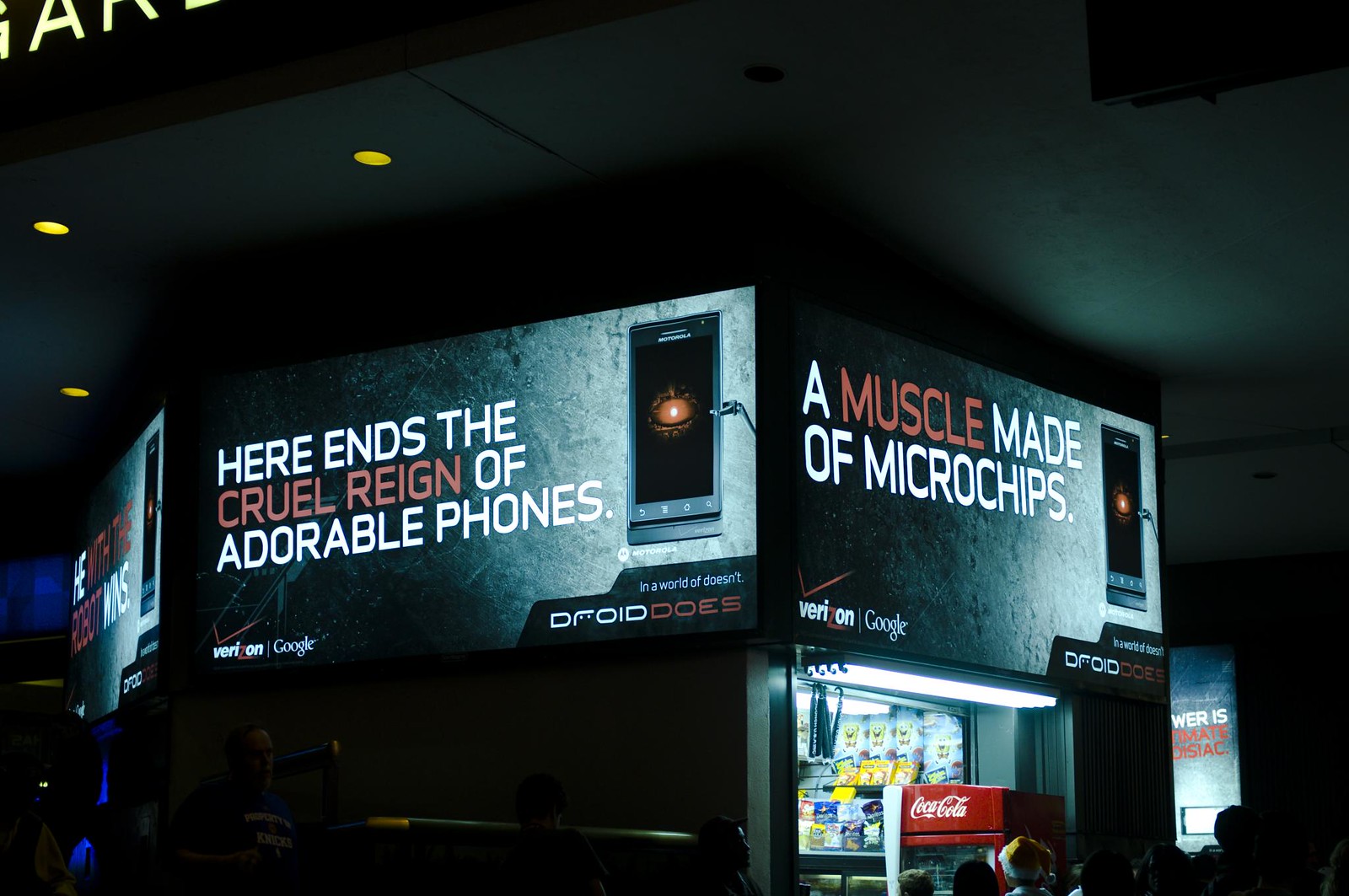This nighttime photograph captures the exterior of a convenience store, dimly lit but identifiable by the neon lights and a prominent Coca-Cola vending machine placed outside. The setting gives the impression of being either under a stadium awning or within a venue with several kiosks. The focal point of the image, however, is the large advertisement painted on the walls above the store. 

On the right side, the ad reads, "A muscle made of microchips," featuring an image of a mobile phone, identified as a Droid, with "Verizon" and "Google" logos and the word "Droid" in the lower right-hand corner. On the left, the ad declares, "Here ends the cruel reign of adorable phones," again highlighting both Verizon and Google in the lower left-hand corner and reaffirming "Droid" in the lower right. The slogan "In a world of doesn't, Droid does" underscores both sections of the ad. The predominant green color of the advertisement contrasts with the dark surroundings, making it the dominant visual element in the image.